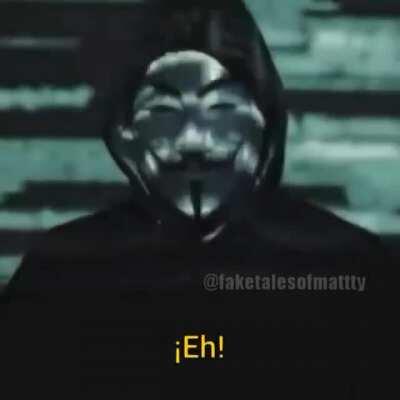The image depicts a character that looks like a scene from a horror movie. The character is wearing a black outfit with a hood, and a stark white mask that portrays an almost eerie Asian-inspired face. The mask features distinct black eyebrows, a handlebar mustache that curves straight upwards, slits for eyes, and a small triangular goatee, also described as a black soul patch. The background of the image is composed of blurred shades of gray, suggesting either a dimly lit room or a monochromatic setting. In the bottom center of the image, the text "¡EH!" appears in a bold yellow color, with an upside-down exclamation point at the beginning and a right-side-up exclamation mark at the end. Additionally, a watermark reading "At Fake Tales of M-A-T-T-Y" is present in light gray text on the darker background. This watermark may also appear differently interpreted in context as "Fake Tails of Maddie" or "fakes tales, full muddy."